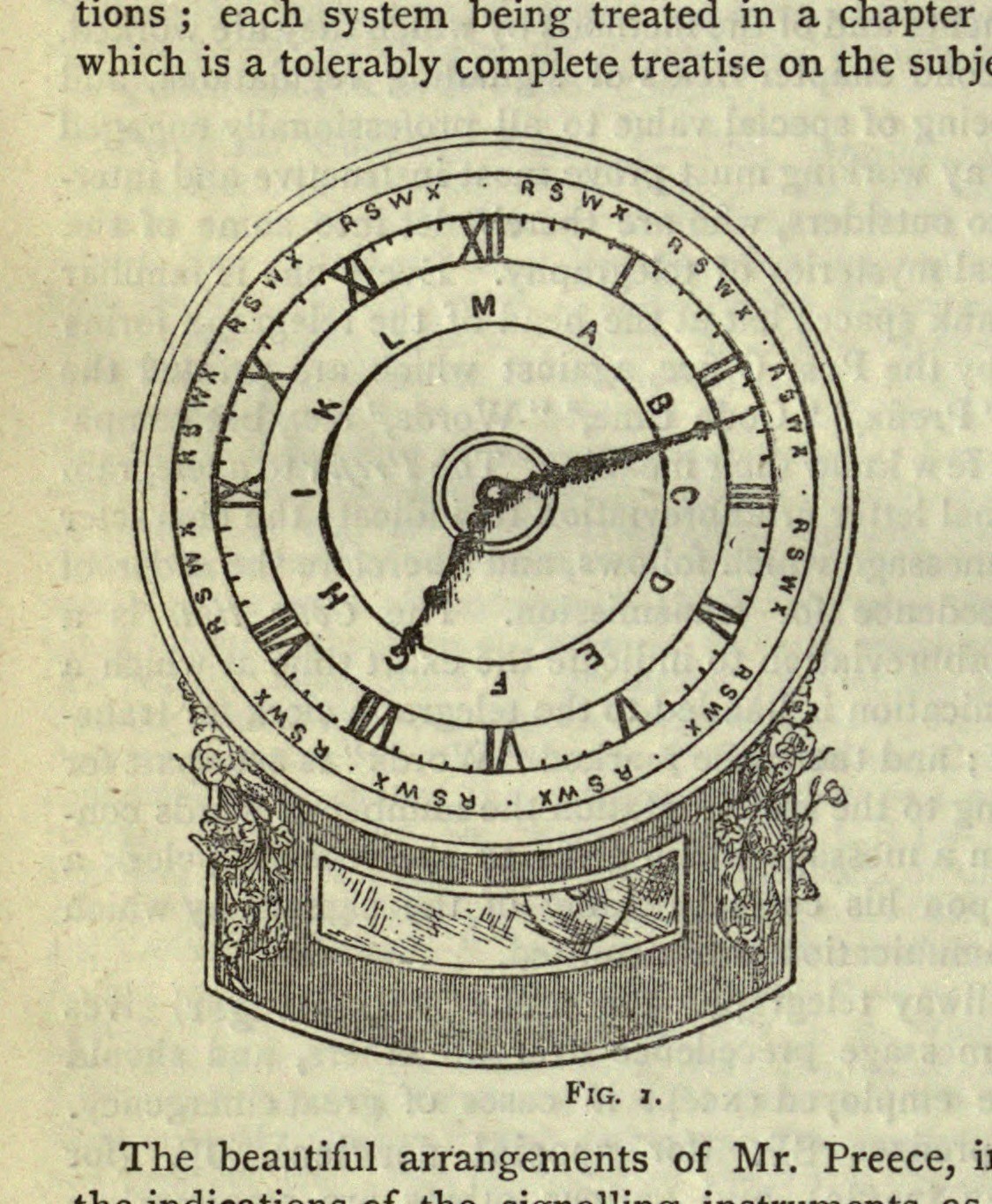This detailed black and white line drawing, likely derived from a woodcut or etching, showcases an ornate clock. The clock, presented in a style reminiscent of a textbook illustration or newspaper print, features a vertically striped base with a window revealing a swinging pendulum. The base is adorned with slight floral designs on either side. The clock face is marked by Roman numerals from 1 to 12, with inner circles containing the letters A through M and an outer circle that repetitively features the letters R, S, W, and X around its border. The clock’s hands currently point to approximately 12 minutes past 7. At the top of the image, partially obscured text suggests it is part of a chapter dedicated to explaining various systems, while the bottom caption reads, "The beautiful arrangements of Mr. Preece, figure 7."